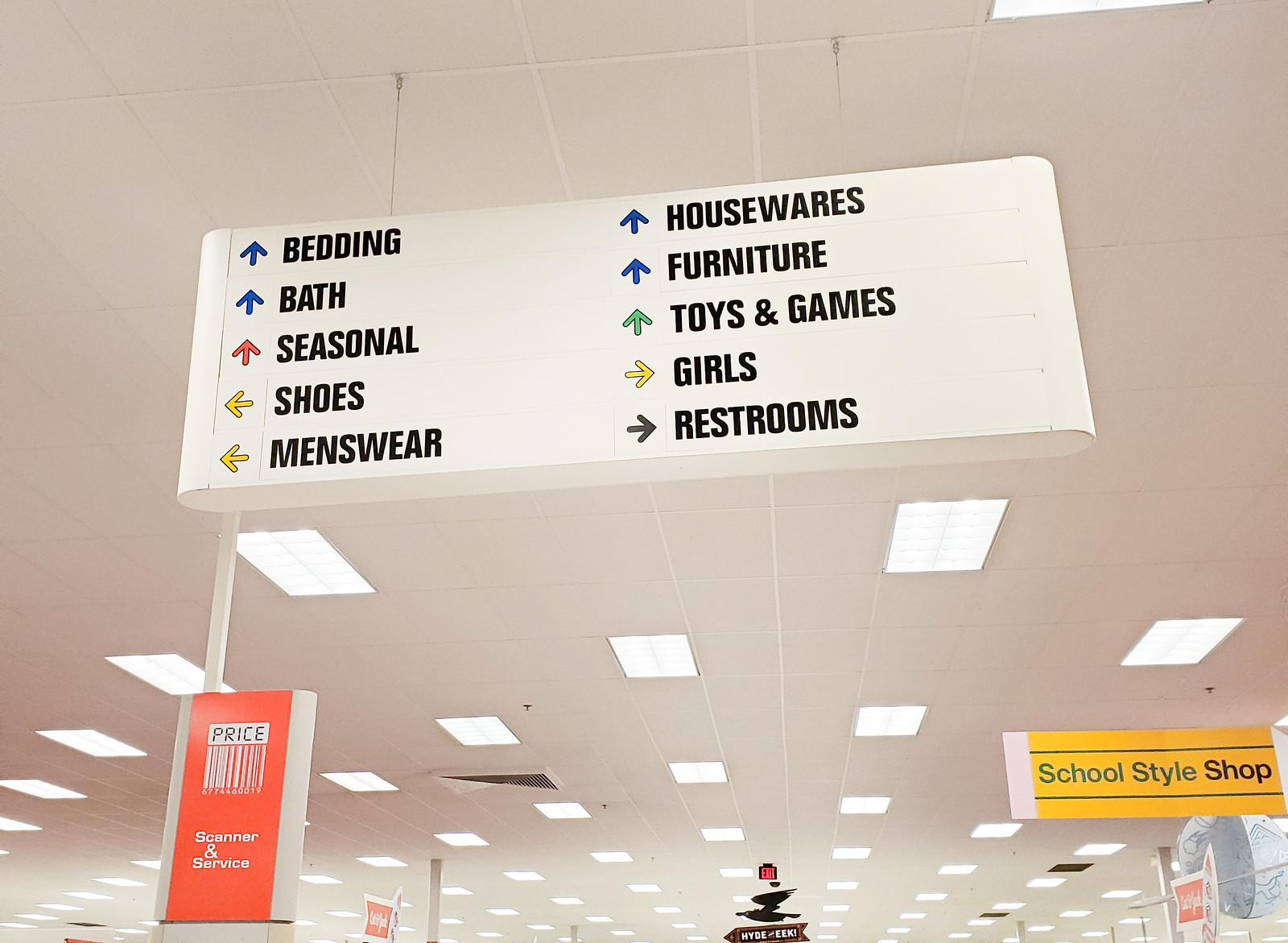This is a color photo taken from a lower angle, looking up at a large directional sign inside a retail store, with focus on the ceiling. The sign displays various store departments with colorful arrows guiding the way: Bedding and Bath, both with blue arrows pointing up; Housewares and Furniture, also with blue arrows pointing up; Seasonal with a red arrow pointing up; Shoes and Menswear with yellow arrows pointing left; Toys and Games with a green arrow pointing up; Girls with a yellow arrow pointing right; and Restrooms with a black arrow pointing right. Additional signs at the bottom of the image indicate a "price scanner and service" area with a red rectangle, and a "school style shop" with a yellow rectangle. The white drop ceiling features numerous fluorescent lights, and there is also a visible misplaced ceiling tile. An eagle or bird with the words "hide eek!" can be seen at the bottom center of the photo. This composition ensures no products or store aisles are visible, emphasizing the navigation aids in the store's environment.